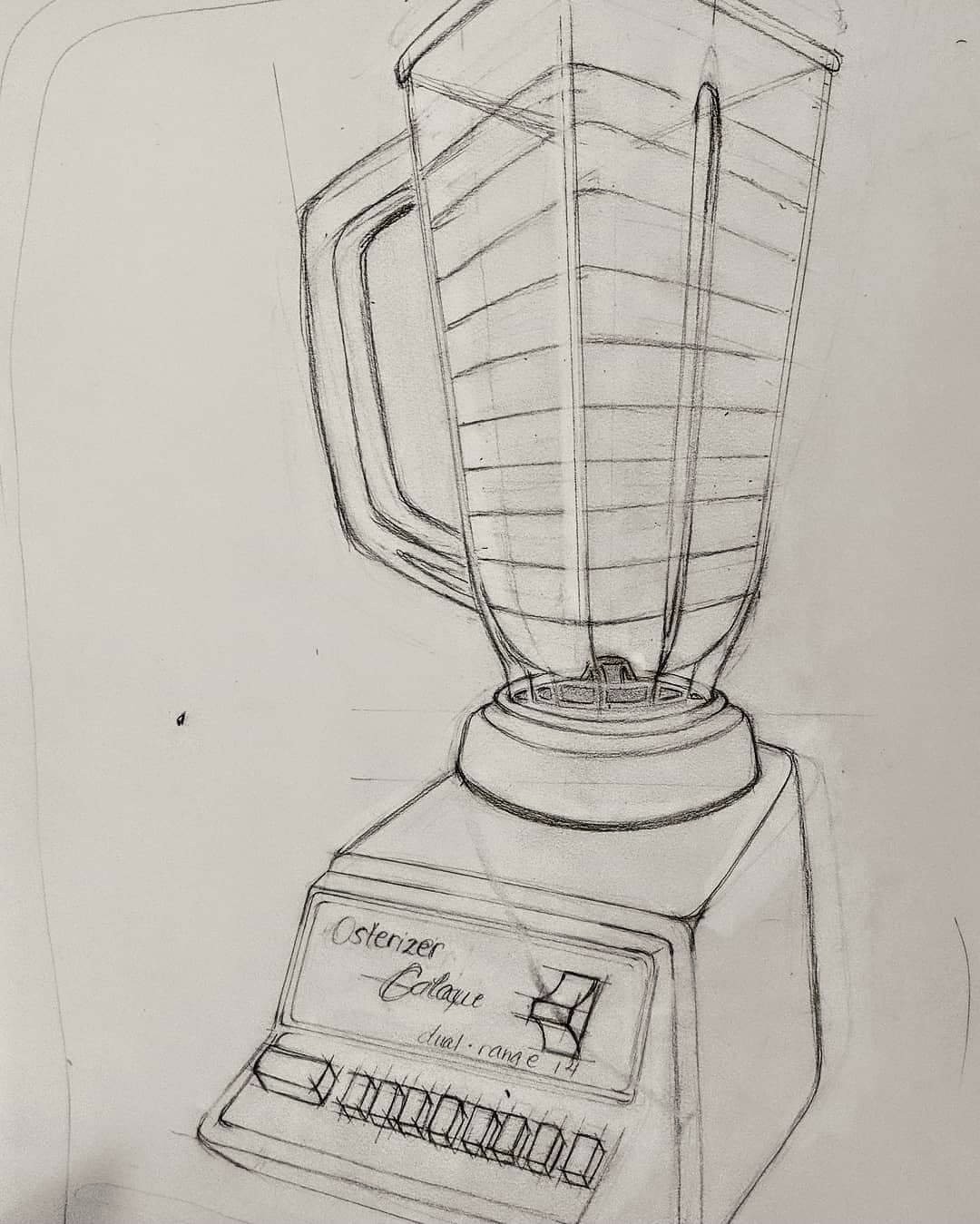This detailed pencil sketch depicts an Osterizer blender with a sturdy, square base. On the faceplate of the base, one can see the clearly written name "Osterizer," followed by a partially obscured word that likely reads "Galaxy." Beneath this, the label "Dual Range 14" is prominently displayed. Below the label, there is a row of control buttons, featuring a wider rectangular button first, followed by eight smaller, uniformly-sized buttons. Atop the base sits a glass bowl with distinct measurement lines etched vertically along its sides, adding both functionality and aesthetic detail to the classic kitchen appliance.